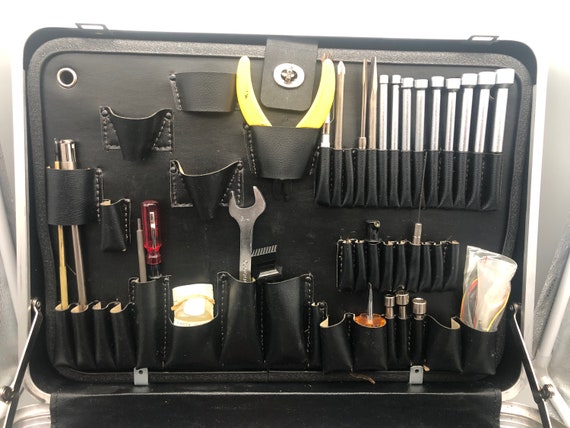This photograph showcases the inside of a heavy-duty, black tool case that's propped open, revealing the top half of the organizer. The interior features a meticulously organized arrangement of black leather pouches stitched onto a black backing. The various compartments hold an assortment of tools typically used by mechanics, handymen, or electricians. Prominent among these are screwdrivers, pliers with yellow handles, a silver wrench, and various wrenches and spanners. There are specific areas designed for different types of tools, including conical pockets and narrow slots for smaller bits and fasteners. Noteworthy is a ziplock bag containing black, red, and yellow cables, hinting at its possible use for electrical work. The metal brackets and hinges are visible, indicating the sturdy construction of the case. The surrounding background is somewhat obscured by a grayish cloth, directing full attention to the meticulously housed tools.